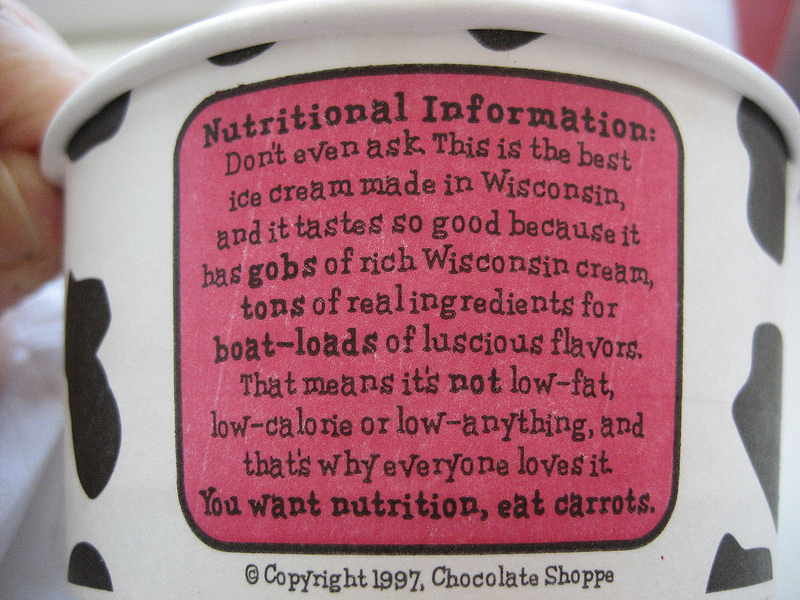In the image, a grayish background with hints of white and pink on the sides frames a partial view of a person's hand with a few fingers visible, resting on a white surface. Dominating the scene is a large, white cardboard tub adorned with black cow print designs. Behind the tub is a prominent pink circle outlined in black, displaying nutritional information in bold black letters. The text humorously advises against questioning the nutritional content, emphasizing the indulgent quality of the ice cream. The product boasts rich Wisconsin cream and abundant real ingredients, promising a plethora of luscious flavors. It's explicitly mentioned that the ice cream is not low-fat, low-calorie, or "low-anything," underscoring its decadent appeal. A cheeky note suggests choosing carrots for nutritional value instead. The tub is labeled with a copyright from 1997, proudly associated with the Chocolate Shop, renowned for its delectable Wisconsin ice cream.